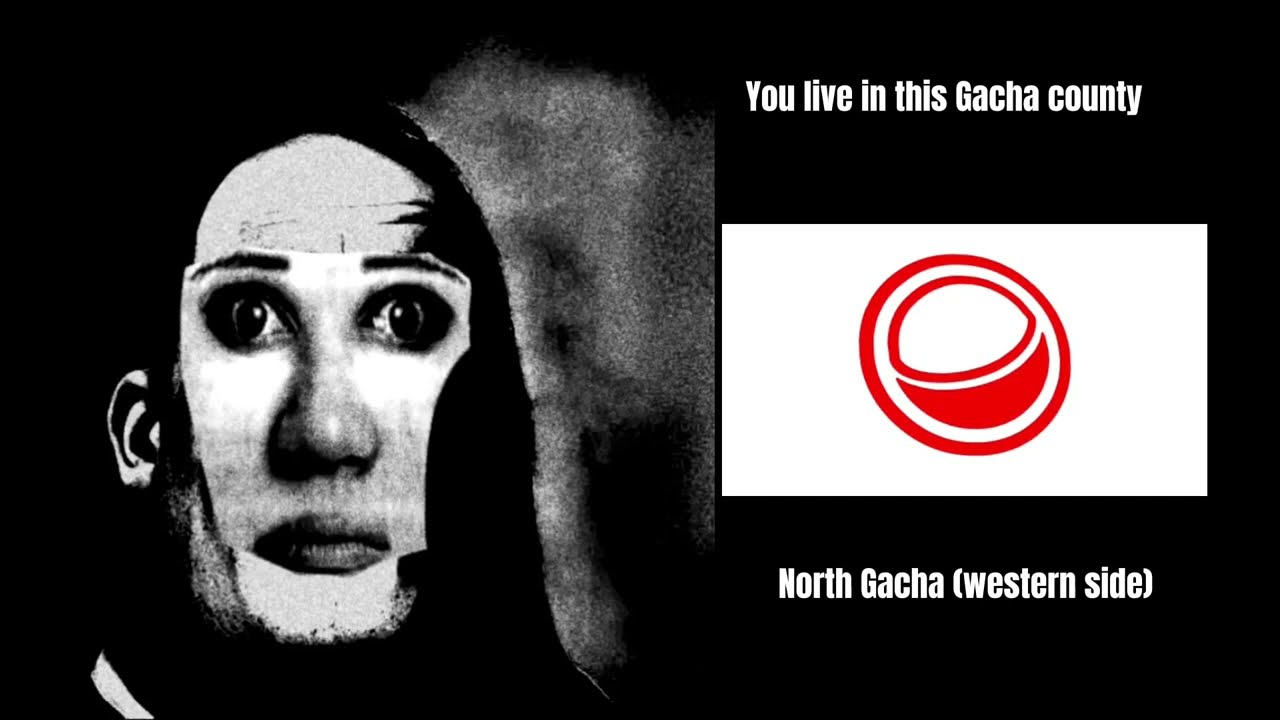The image presents a surreal collage with a black background. On the left side, there is a creepy, manipulated face, likely edited to combine different facial features. The base appears to be a black and white photo, with sections of a woman's lips, wide, bulging eyes accentuated with dark mascara, and a pronounced bulbous nose, making it unsettling. The man has long hair cascading over the sides of his face, and his features are highlighted by various shades of gray.

On the right side, a logo takes center stage. Above it, in vivid white text, the words "You live in this Gotcha County" are displayed prominently. The specific phrasing "Gotcha County" may intentionally or unintentionally create an element of intrigue or mockery. Beneath the logo, the text "North Gotcha (Western Side)" appears, written in the same white font.

The logo itself is within a white box, featuring a circular design that includes a red outer ring, a white crescent, and additional red and white elements creating complex visual symbolism. The whole composition appears as if it's intended for social media, perhaps as a provocative advertisement or artistic statement meant to capture attention through its unsettling and mysterious design.